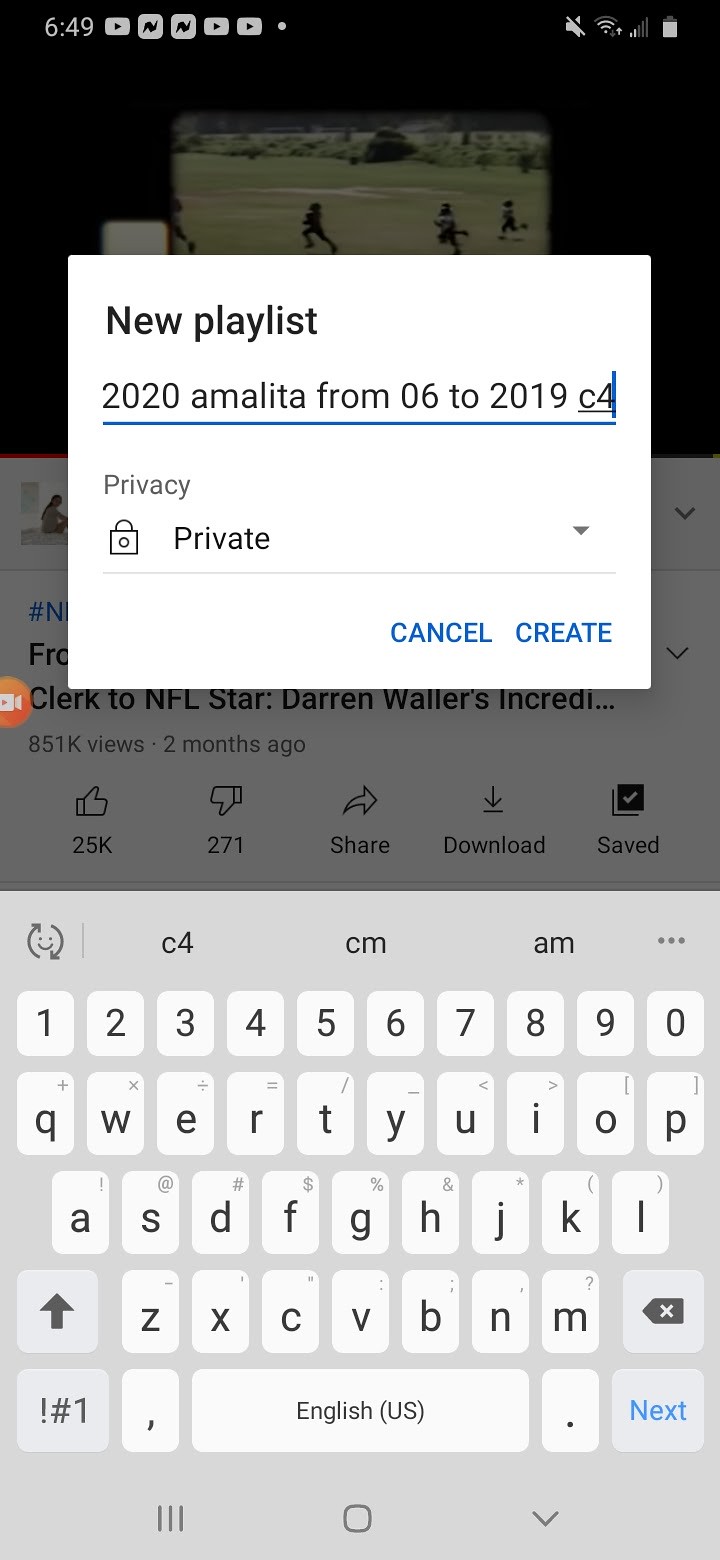The image captures a screenshot of a smartphone display in portrait orientation. At the top of the screen, the status bar indicates the time as 6:49. It shows the absence of Wi-Fi, displays the cellular signal strength, and indicates the current battery level. The main portion of the screen features a translucent overlay with an active pop-up that reads "New Playlist." The suggested playlist title is "2020 Amelita from 06 to 219C4." Beneath this input field, there is an option to set the playlist to "private," and buttons labeled "Cancel" and "Create," both of which are unselected.

The background reveals a paused video that appears to cover a sports event, likely a football game, showcasing what seems to be a player running down a field being pursued by an opponent. The partially visible text from the video suggests a headline or description, reading "Clerk to NFL star Darren Walters in cred," hinting at its sports-related content. The video is hosted on YouTube and has garnered 851,000 views.

At the bottom, the standard smartphone keyboard is visible, providing input capabilities for the user. Altogether, the screenshot presents an interface where the user is in the process of creating a new playlist while watching sports content on YouTube.